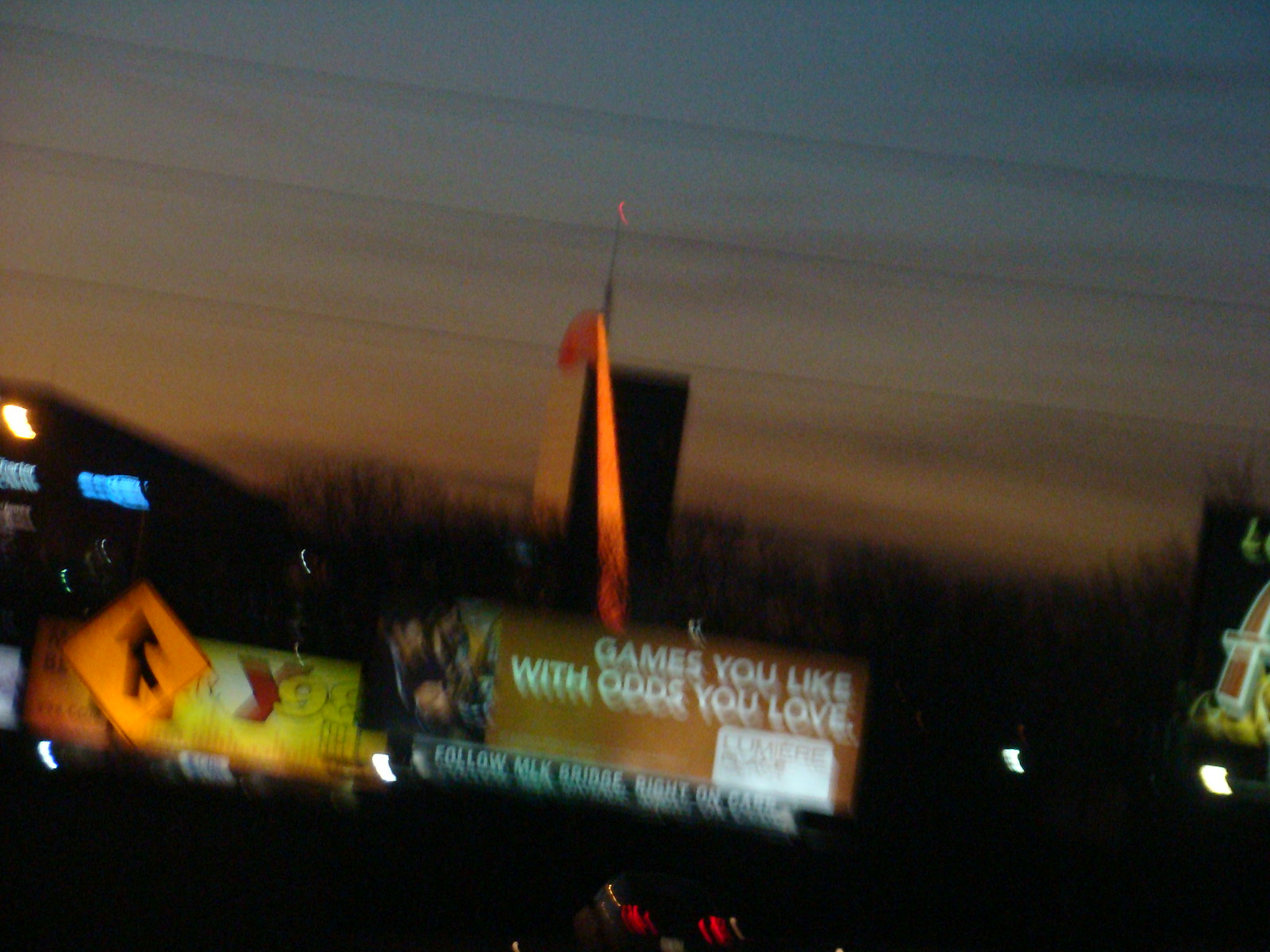A nighttime cityscape photograph captures a couple of billboards and buildings, all enveloped in a blur that gives the image a double exposure effect. The primary focus is a prominent billboard featuring a yellowish-orange background with the text, "Games you like with odds you love," in white letters, although the text appears indistinct and doubled due to the blurriness. Below this slogan, another line reads, "Follow MLK Bridge, right on car," set against a darker background in crisp white letters. 

To the left, partially obscured by a road construction sign displaying an upward arrow in an orange diamond, another billboard emerges, but its details remain indiscernible. In the same area, part of a building exhibits faint neon lettering, hinting at a store or establishment, though the specific wording is lost in the blur. On the right side of the photo, another billboard is barely visible, not revealing enough to identify its content.

Above, the night sky features an intriguing blend of dark gray with streaks of orange, adding to the photo's surreal ambiance. The outline of a rectangular building stands against this sky. Below the main billboard, what appears to be the blurred taillights of a vehicle add another layer of motion and light to the scene. The entire composition evokes a sense of urban chaos and nocturnal beauty, seen through a hazy, dreamlike lens.